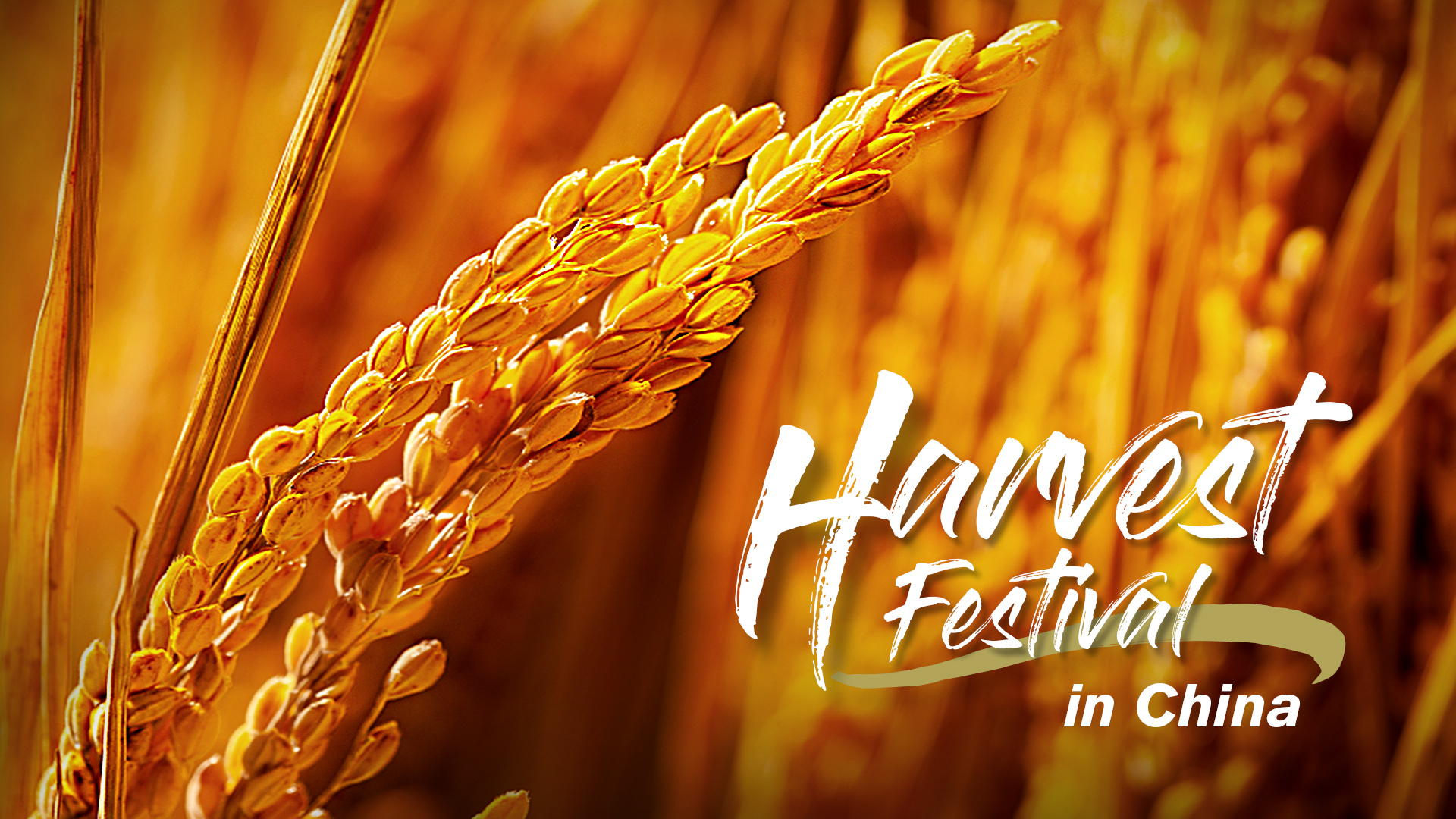The image is a wide poster titled "Harvest Festival in China," featuring a photograph that has been edited to include golden and golden-brown tints, giving it the warm hues of a sunset. Dominating the left side of the poster is a prominently displayed, highly detailed stalk of wheat that curves toward the center. The backdrop includes more wheat plants, but these are blurred, highlighting the main stalk in the forefront. The text "Harvest Festival in China" appears in stylized white font on the bottom right, entirely in English, which is somewhat unusual for a poster about a Chinese festival. The overall appearance of the poster, with its rich gold tones and detailed wheat images, raises curiosity about whether the plant is computer-generated. This meticulously designed poster seems to be aimed at an English-speaking audience, possibly for educational purposes to introduce the concept of a harvest festival in China.